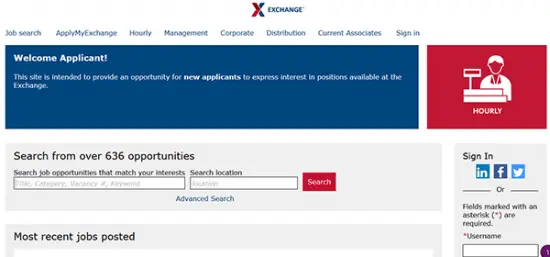The website features a clean, white background with a prominent 'X' design in the center. The left side of the 'X' is red, while the right side is blue, and the word "Exchange" is displayed in blue text across the middle. 

The left-hand side hosts a blue tabbed menu labeled "Job Search," which includes options such as "Apply My Exchange," "Hourly Management," "Corporate," "Distribution," and "Government and Social Services." Below this, a blue rectangle contains white text saying "Welcome Applicant." A statement informs new applicants that the site is intended to help them express interest in positions available at the exchange. 

A red-bordered rectangle features an icon depicting a person at a cash register. In a white space beneath this, black text reads, "Search from over 636 opportunities," followed by "Search job opportunities that match your interests." Below, there are fields labeled "Search Location" with corresponding text boxes beneath each.

To the right of these fields, a red and white button is labeled "Search." Below the search button, blue text reads "Advanced Search." 

On the right side of the webpage, there is a gray box with black text stating "Sign In," alongside LinkedIn, Facebook, and Twitter symbols. The word "OR" appears, followed by the instruction, "Fill Mark With An Easy Access of Required Username," in black text. A text box below this area is provided for users to type in their username.